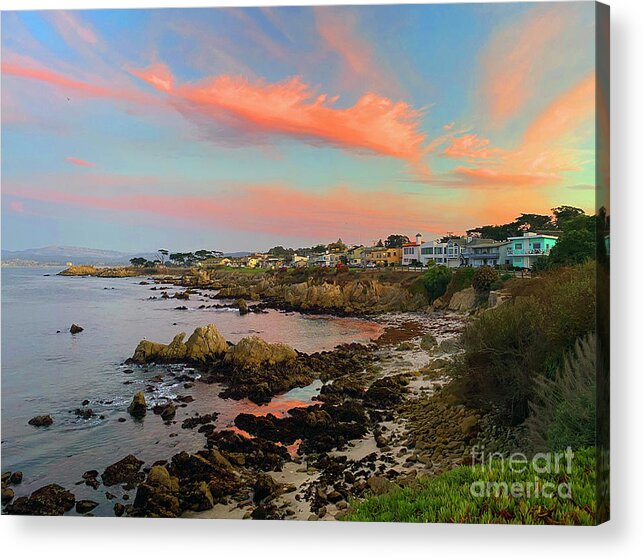The photograph depicts a beautifully detailed painting or highly realistic photograph of a coastal landscape. The top half of the image features a bright blue sky adorned with pink-tinged clouds, suggesting a sunrise or sunset. Below, the scene is divided into two main sections: the left side showcases a body of water with rocky formations and some rocks extending into the water. The right side features a rocky shoreline with patches of sand and abundant greenery, including grass, weeds, and bushes. The land curves out towards the center of the image, gradually leading into a picturesque waterfront community. Around 20 houses of various colors—white, yellow, and red—line this coastal stretch, though they are distant enough that individual details aren't prominent. The vivid and well-lit scene appears to capture natural sunlight, enhancing its clarity and vibrancy. In the bottom right-hand corner, the text "Fine Art America" is inscribed in white, indicating either the artwork's origin or platform.